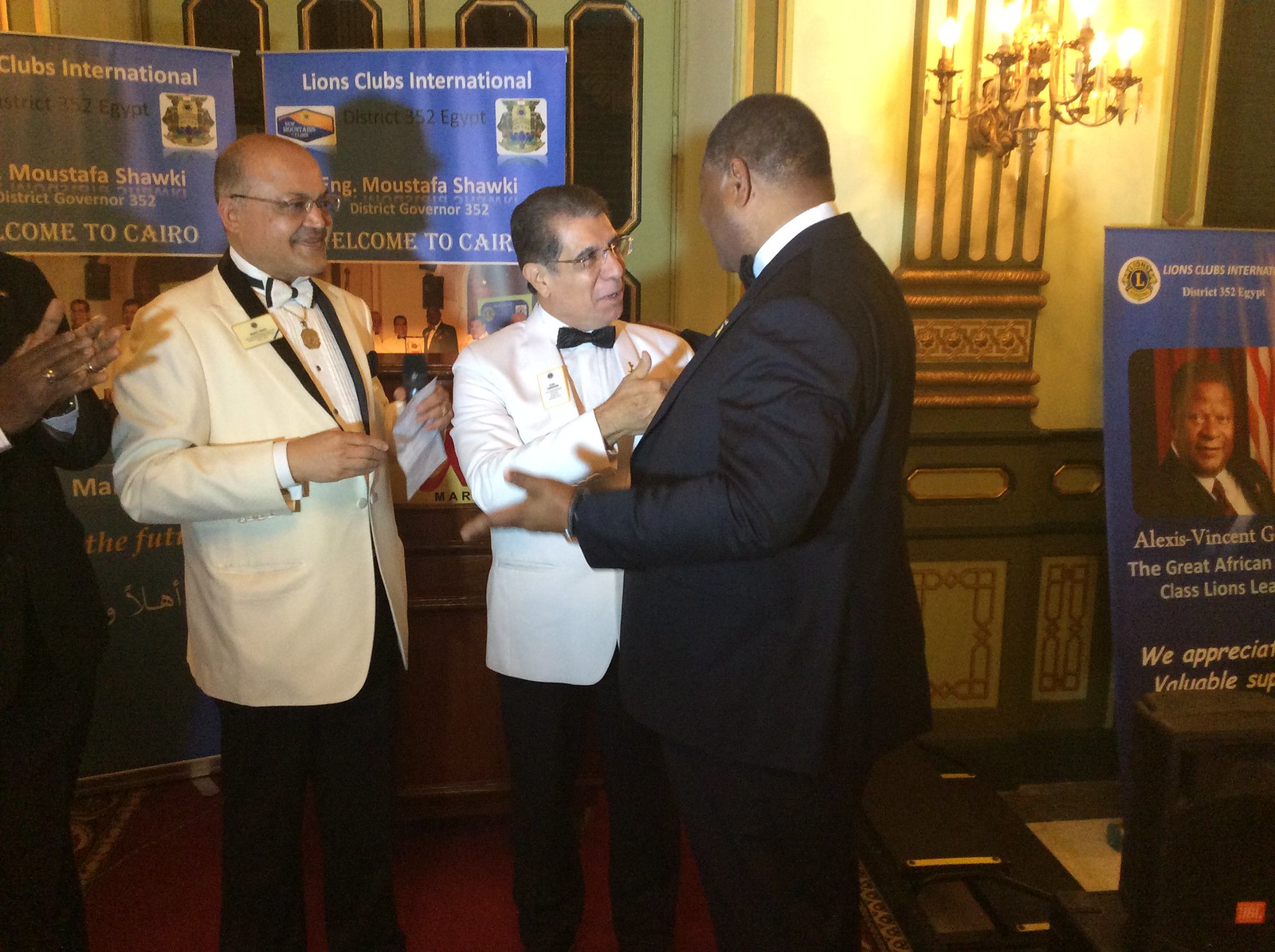In the image, three men are the focus, two of whom are dressed in white jackets and bow ties, paired with glasses and name tags on their jackets. They are engaging in conversation with an African American man on the right, who is dressed in a black jacket and pants, with a glimpse of a white button-down shirt visible. The setting appears to be an elegant room, characterized by a chandelier and a wall-mounted candelabra. Various signs adorn the walls, including one that reads "Lions Club International, welcome to Cairo." Another poster to the right of the man in the black suit prominently displays his face against a blue background with white text. In the background, partially obscured, a person is clapping, suggesting a ceremonial event, possibly an award presentation or recognition. The detailed ambience and interactions hint at a formal, celebratory occasion.